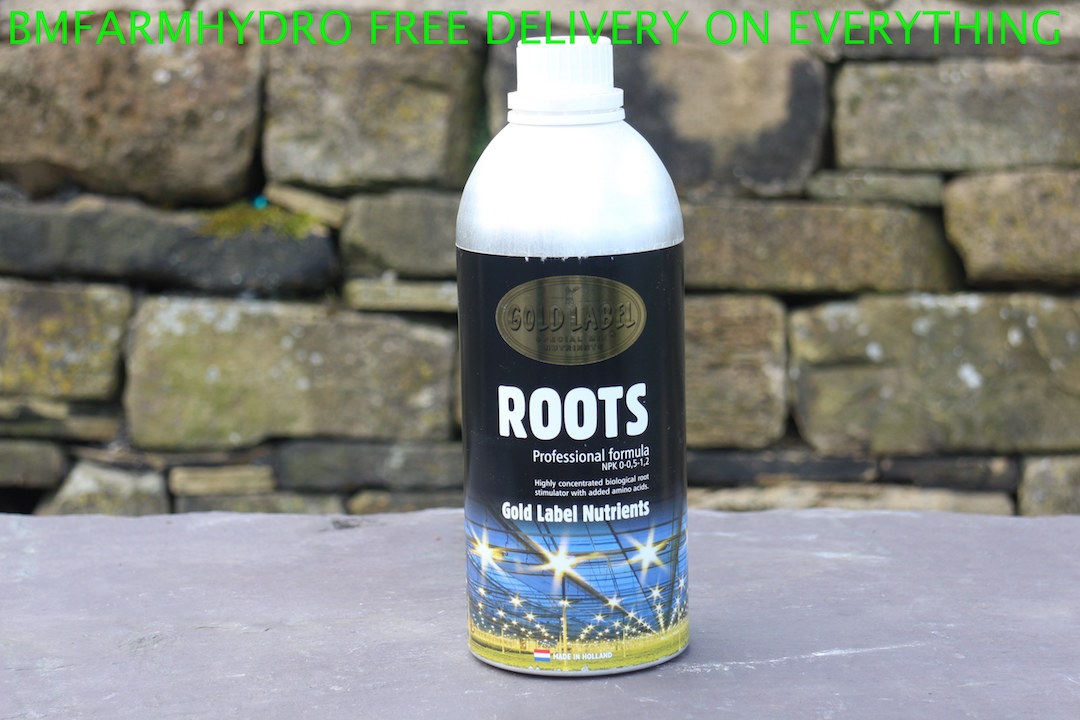This image is a detailed photograph of a nutrient product in a white plastic bottle with a white cap, prominently positioned on a stone or concrete slab, possibly outdoors. The background showcases a stone wall that is partially covered with moss and lichen, reinforcing the outdoor setting. At the top of the image, there is horizontal text in neon green, displaying the message: "B.M. Farm Hydro, free delivery on everything" in all caps. 

The bottle itself features a large black label that transitions into a blue and yellow design towards the bottom. There's a distinctive gold oval at the top of the label that reads "Gold Label." The main text on the bottle includes "Roots" in large white letters, followed by "Professional Formula" and "Gold Label Nutrients" in smaller letters. The label also mentions that it contains a "Highly Concentrated Biological Root Simulator with added amino acids," suggesting its use for plant nutrition. The bottom part of the label appears to show an image of a large factory or farm, which may allude to the product's industrial or professional-grade quality.